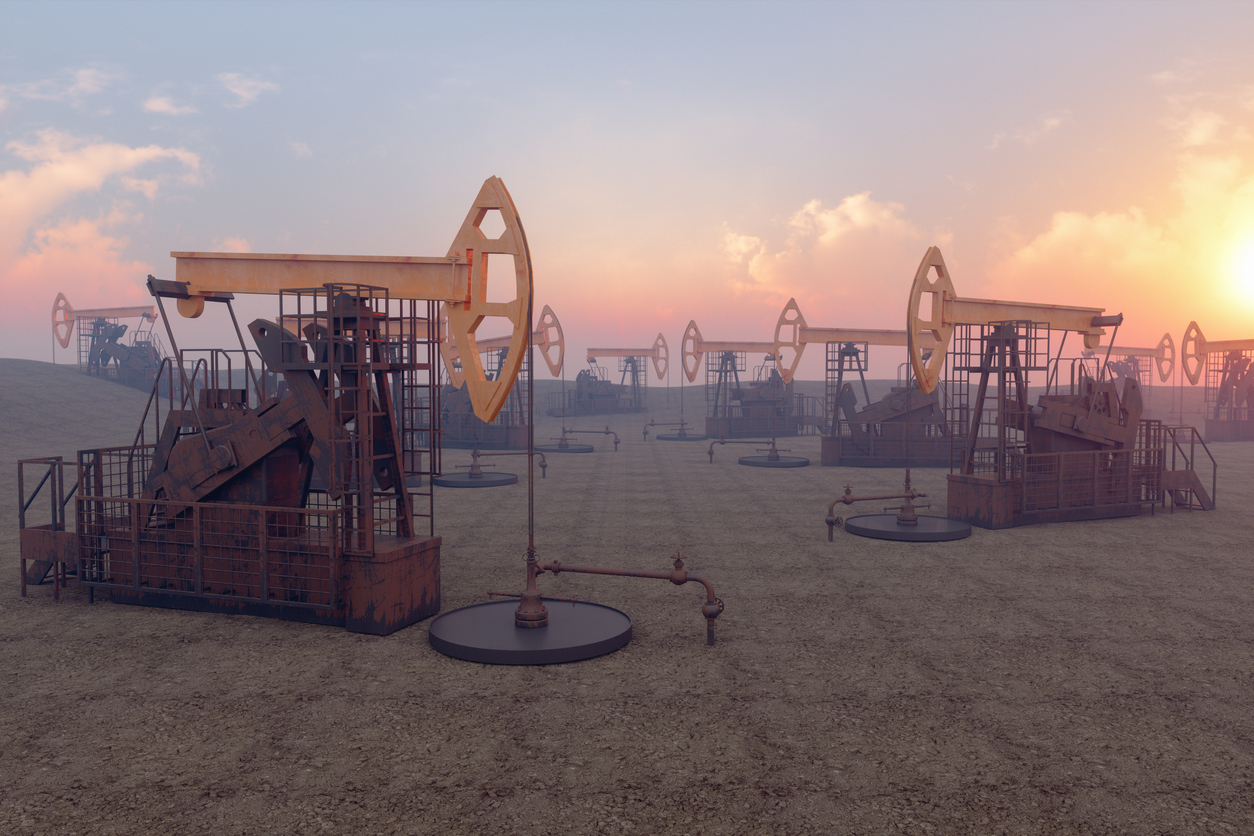The photograph captures an industrial oil field at either sunrise or sunset, marked by the striking colors of the sky. The top of the sky features a darker blue and purplish hue, transitioning to an array of pink, purple, and yellow as it descends, with the sun peeking out from the right side of the image. The scene is set against a hazy backdrop, with colorful clouds scattered throughout.

The ground below is composed of reddish-brown dirt a with grid-like pattern, almost barren and rocky. Dominating the field are several oil rigs, organized in rows that stretch from the front to the back and side to side of the image. These rigs feature rust-colored bases and large yellow drilling arms, resembling erector-set constructions or giant keys. Each rig is connected to the ground through pipes ending in black circular plates.

There are at least nine visible oil rigs, with some estimates suggesting up to eleven, each appearing identical in structure. The photo vividly captures the mechanical uniformity of the equipment against the natural beauty of the transitioning sky.